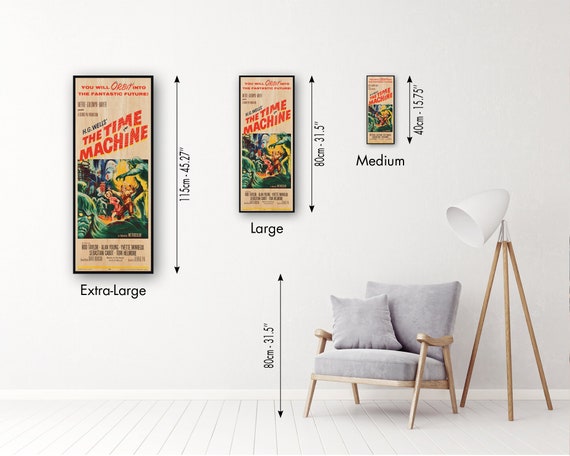This is a meticulously staged advertisement photo shot indoors with an emphasis on clarity and product display. The room features pristine white walls and white wooden panel flooring. Centrally positioned is a light oak chair adorned with a gray cushion. Adjacent to the chair is a matching light wood tripod lamp with a cone-shaped white shade that illuminates the scene. Prominently displayed on the wall are three identical posters for the movie "The Time Machine," each available in three different sizes: medium (40 centimeters), large (80 centimeters), and extra large (115 centimeters). Each poster is accompanied by labels and dimensions, illustrating how far each size hangs from the floor, likely to help potential buyers visualize the scale and placement. The setup resembles a catalog image, akin to what one might find on Etsy, showcasing both the artwork and furnishings in a cohesive, minimalistic setting.